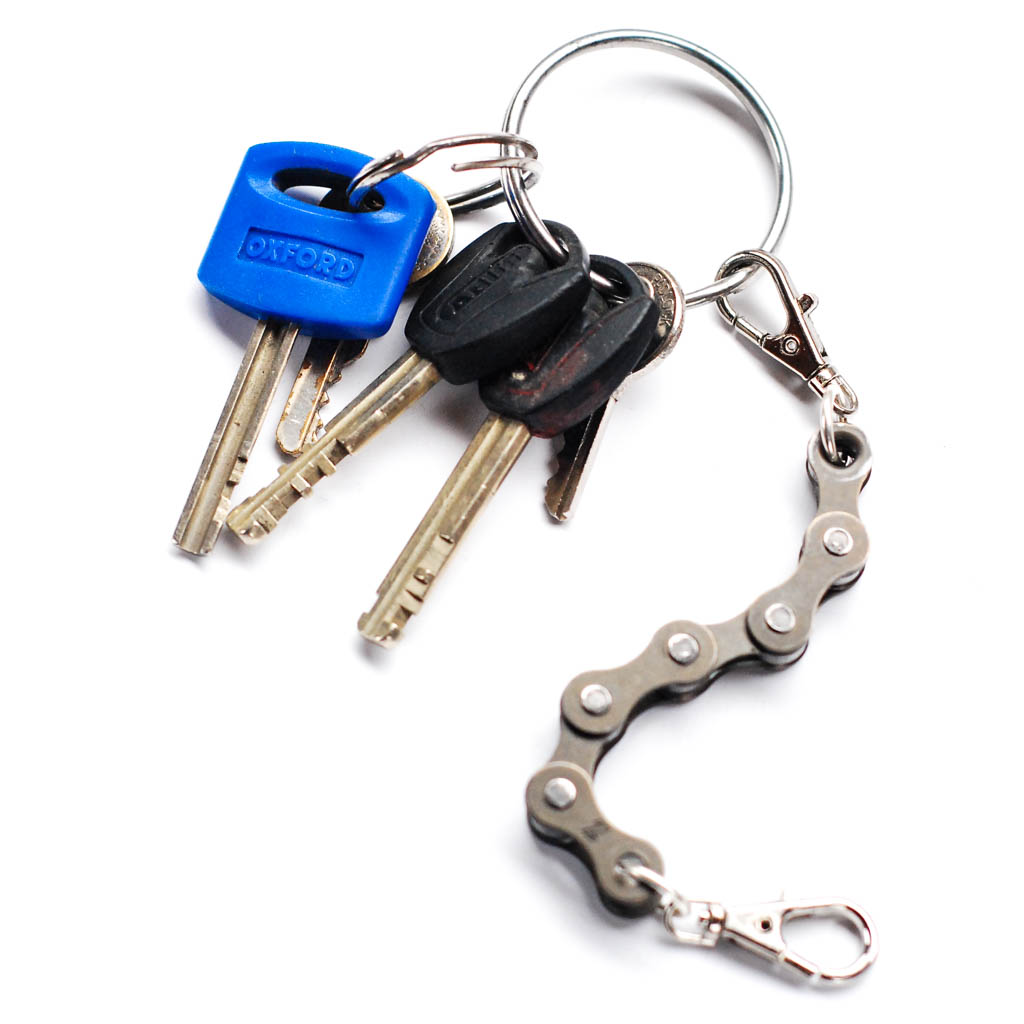This image depicts an assortment of keys on a metal keychain, situated on a white background. The keychain features five keys in total. Among them, two keys have black plastic casings on their heads, while two others are devoid of any plastic covering and remain entirely metallic. One key stands out with a blue plastic covering engraved with the word "OXFORD" in uppercase letters. In addition to the keys, there's a distinctive keychain accessory attached, resembling a bicycle chain with visible steel rivets and a metal clasp, which could be used to hook onto various items. The entire setup, including the keys and keychain elements, appears to be slightly worn, suggesting it might be an image taken indoors on a white table, possibly related to a lost and found item.